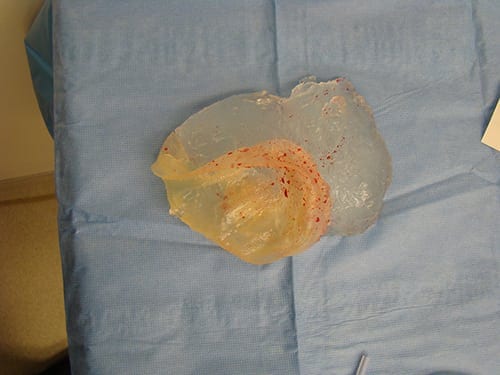The photograph depicts an unknown glutinous mass resting on a bluish-white surface, which resembles a medical sheet or thick bandage, potentially tissue paper. Central to the image is the mysterious object, exhibiting a jellied appearance. The mass predominantly features a clear, reversed L-shaped section, accompanied by surrounding areas of varying hues including orange and pinkish-yellow. Among these colored regions, there are small, redder spots that evoke the appearance of blood. Notably, within its left section, a distinguishable, possibly fish-shaped yellow formation is observed, suggesting a different texture. Despite its detailed appearance, the precise nature of the object remains unidentified, though it might be speculated as a removed implant, potentially of silicon origin.